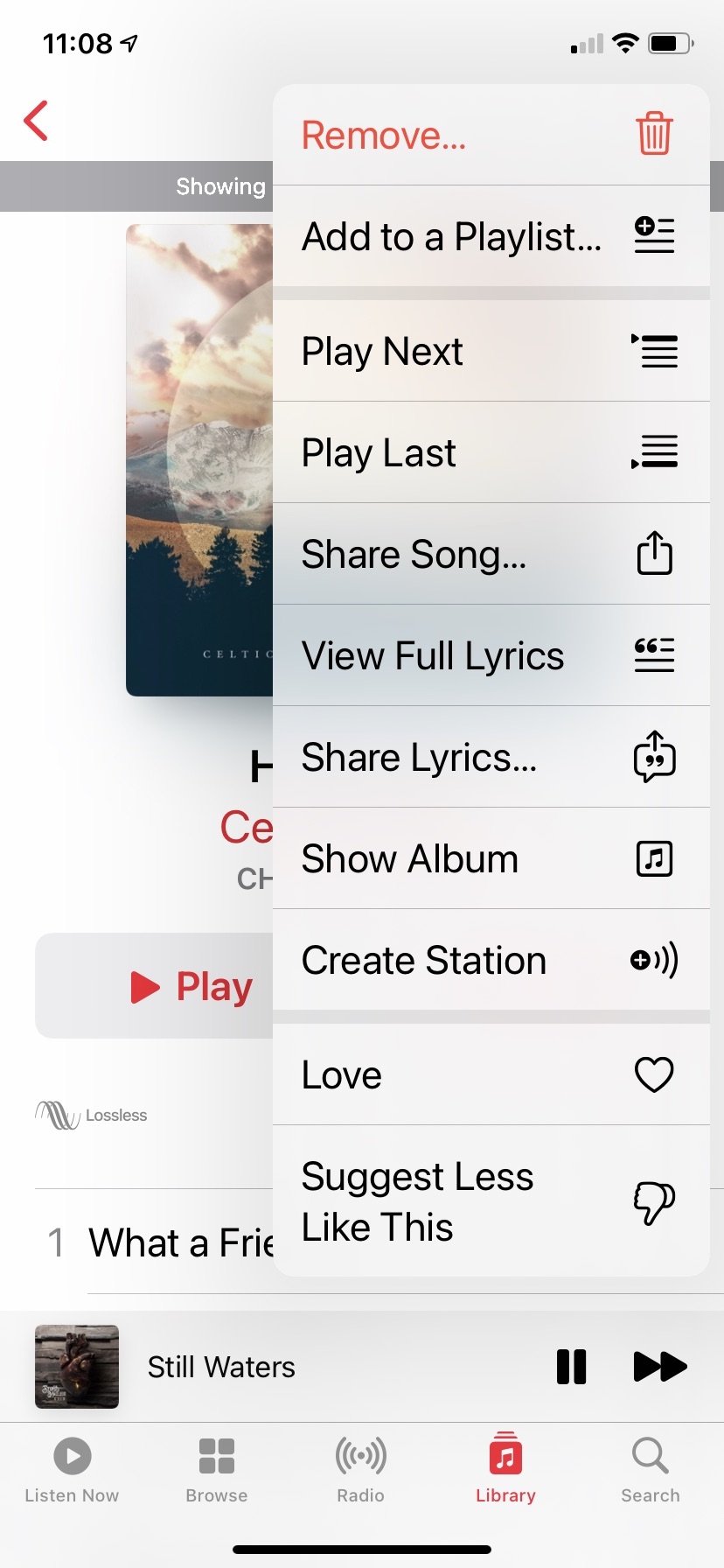This is a detailed screenshot from a cell phone, showcasing both the phone's screen and a superimposed pop-up menu of options. 

Starting with the main screen in the background, it is 11:08 AM, as indicated at the top. The status bar on the right displays one out of four signal bars, an active Wi-Fi connection, and a battery that's approximately three-quarters full. Below this status bar, there is a playlist interface. A gray bar at the top contains the word "Showing" in white font. Beneath this, there is a visually striking graphic of a full moon partially obscured by purple and yellow clouds, positioned above a silhouetted landscape of evergreen trees.

Directly under this graphic, there is a red "Play" label accompanied by a red play button. Moving further down, the song "What a Friend" is displayed, along with associated details. The album cover of "Still Waters" appears on the left, and on the right side, there are standard playback controls: a pair of side-by-side vertical rectangles representing the pause button, and two black, touching arrows for the fast-forward button.

At the very bottom of the screen, there are five navigation commands: 
1. "Listen Now" under a circle with a white arrow, 
2. "Browse" represented by four small rectangles arranged in two rows, 
3. "Radio" iconified by radio waves,
4. "Library," which is currently selected and highlighted in red, depicted as a box containing two white music notes, 
5. "Search" represented by a magnifying glass.

The pop-up bar, which is narrower and overlaid on the main screen, features several options. At the very top, it says "Remove" in red text, accompanied by a red garbage can icon, indicating it is selected. The subsequent options are listed in black font with corresponding icons: 

- Add to playlist
- Play next
- Play last
- Share song
- View full lyrics
- Share lyrics
- Show album
- Create station
- Love (with a heart icon)
- Suggest less like this (indicated by a hand with the thumb pointing downward)

Icons for playback variations generally show horizontal lines with different ones emboldened. Each option corresponds to a typical function seen in music streaming apps.